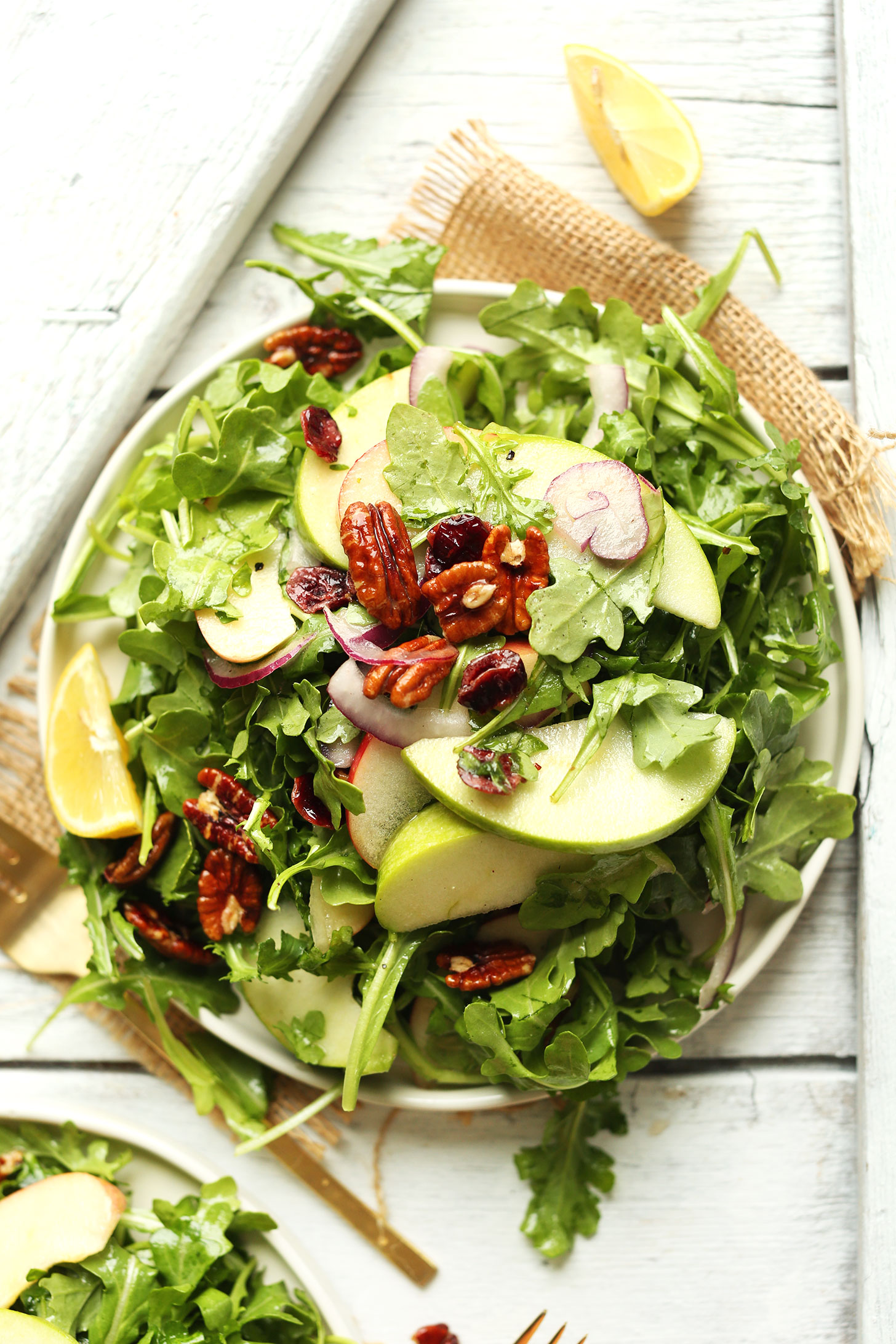The overhead photograph showcases an elaborate rustic salad presented in a shallow, round white bowl with a slight upper lip, positioned atop a piece of burlap serving as a placemat. The setting is a white wooden tray shaped like a triangle, placed on a backdrop of whitewashed wooden planks. The salad is a vibrant mix of leafy greens including arugula, spinach, and possibly other mixed greens. Adorning the salad are thin slices of both green and red apples, adding a touch of color and texture. Scattered throughout are candied walnuts and dried cranberries, providing a sweet contrast. There are also pecans and perhaps bits of red onion or radish hearts, enhancing the visual and flavor complexity. The entire salad glistens with a light vinaigrette dressing. Nestled within the salad are wedges of lemon, with additional lemon slices placed alongside the gold fork that accompanies the dish. In the background, a slightly cropped additional salad bowl or plate can be seen, hinting at a shared meal.